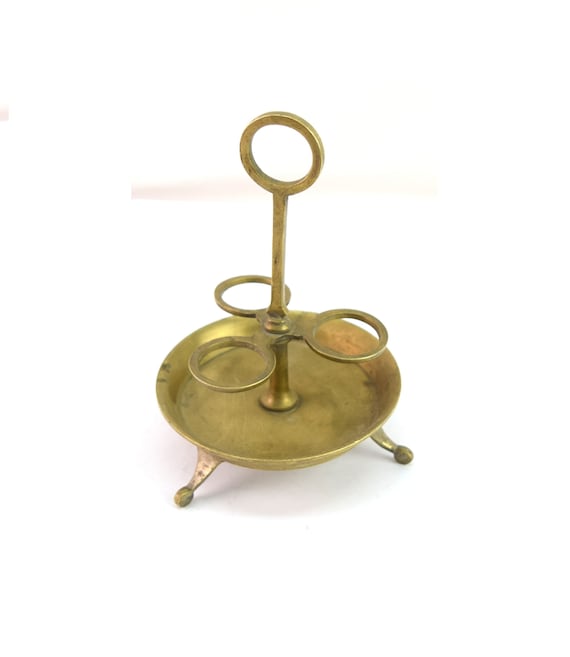This close-up image showcases an antique brass piece, likely a candle holder or a decorative stand. The brass object features three small feet at its base, supporting a shallow circular dish marked with signs of age and wear. Centrally positioned on the dish is a vertical stem, which extends upwards, ending in a key ring-style handle for easy carrying. Around three-quarters of the way up this stem, three evenly spaced rings encircle it, each with a small hole that appears to hold decorative items or tall candlesticks. The piece exudes a vintage charm with its weathered brass and intricate design. The stark white background of the image further accentuates the antiquity and the detailed craftswork of the object.